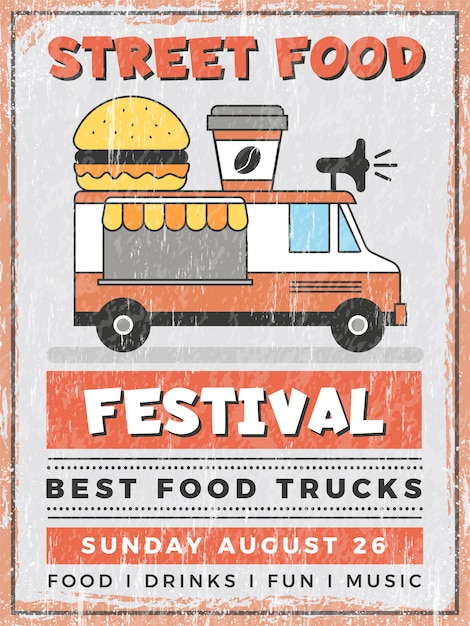This vintage-style advertisement poster promotes a Street Food Festival and features a colorful, clip-art-like image of a food truck. The poster has a deliberately aged appearance with scratchy, weathered paint textures that add to its retro charm. At the top of the poster, "Street Food" is boldly written in red text. Below this, a detailed illustration of a food truck is prominently displayed. The food truck, viewed from its right side, boasts red and white stripes and has a large burger and a coffee cup perched on its roof. Additionally, a bullhorn is attached to the front of the roof, giving it an old-fashioned announcement vibe. The truck’s window, with an awning decorated with yellow and orange doilies, is ready to serve customers their orders. Beneath the food truck illustration, the word "Festival" is showcased in white text within a red rectangular box. Further down, the poster details: "Best Food Trucks" in black text, followed by "Sunday, August 26" in white text within another red rectangular box. At the very bottom, "Food, Drinks, Fun, Music" is listed in black text. The poster is bordered by a reddish-brown frame with an additional black border inside, further emphasizing its nostalgic feel.